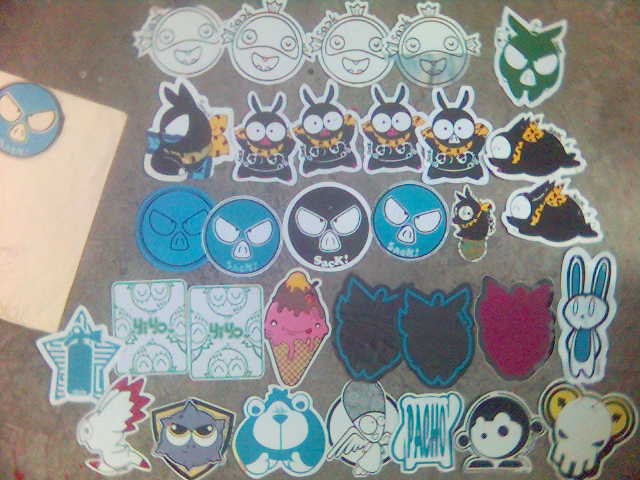The image is a detailed landscape photograph depicting five rows of colorful custom stickers arranged on a brown carpet. The top row features fish stickers, each facing forward with what seems like a crown on their heads. To the right of this row, there's a distinctive green sticker resembling an angry skull with ears and possibly a bandana. The second row consists of bunny stickers with round eyes, and includes two additional bunny stickers in profile positioned on either end, with one lying on its side. The third row showcases four circular face stickers, three in blue and one in black and white, bearing the word "SACK" at the bottom, followed by two more bunny stickers. The fourth row includes a variety of stickers: green ones, a pink ice cream cone with a smiley face, and two or three silhouette stickers, some black outlined in blue and one in pink, ending with a white and blue bunny sticker. The bottom row features a diverse assortment, including an owl sticker, a shield and spike ball sticker with a face, a blue bear sticker, a black and white flying character, a blue and white Pacho sticker, another black and white character, and a final yellow and white skull sticker. In the top left corner, there's a partially visible round sticker with alien eyes on a cream paper. All these elements create a vivid scene of eclectic and animated sticker designs.